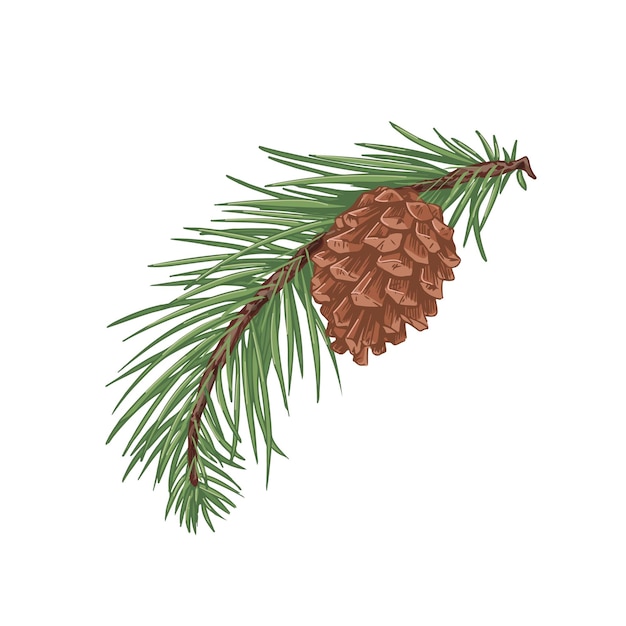This image depicts an illustrated branch of an evergreen conifer, likely a pine or spruce, set against a stark white background. The branch extends from the top right, arching gracefully down to the lower left corner. Detailed pine needles, varying from light to medium green, sprout individually from the brown twig, giving the drawing a textured and lifelike appearance. About a quarter to a third of the way down the branch, a somewhat detailed pine cone, colored in shades of tan and bronze, hangs naturally. The pine cone features intricately shaded scales with small brown dots on their tips, suggesting texture and depth. This simple yet detailed illustration is presented in a style that could easily be suited for educational purposes or digital web use, emphasizing the natural beauty and structure of the conifer branch.